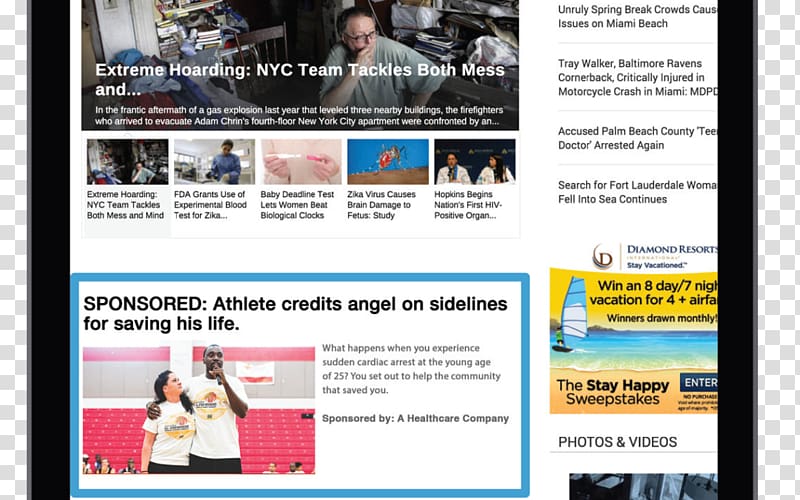This is a detailed screenshot of a news page. The layout features a left and right column of gray and white checks flanking a central black column. At the top of the page, there's a prominent photograph of an older man wearing a t-shirt and glasses. He appears contemplative, with his right hand touching his mouth, and gazes into the distance. The setting around him is cluttered, indicating a messy room.

Overlaying this image is white text that reads: "Extreme Hoarding: NYC Teen Tackles Both Mess and..." Below this main image, there are five smaller pictures, each accompanied by a headline. Additional headlines are positioned to the right of the main photograph.

At the bottom of the page, there's a large advertisement with a blue outline. The ad text reads: "Sponsored Athlete Credits Angel on Sidelines for Saving His Life." The accompanying image depicts a tall African-American man wearing a t-shirt, with his arm around another person who appears to be female. Behind them, red stadium seats are visible, indicating they are likely in a sports venue.